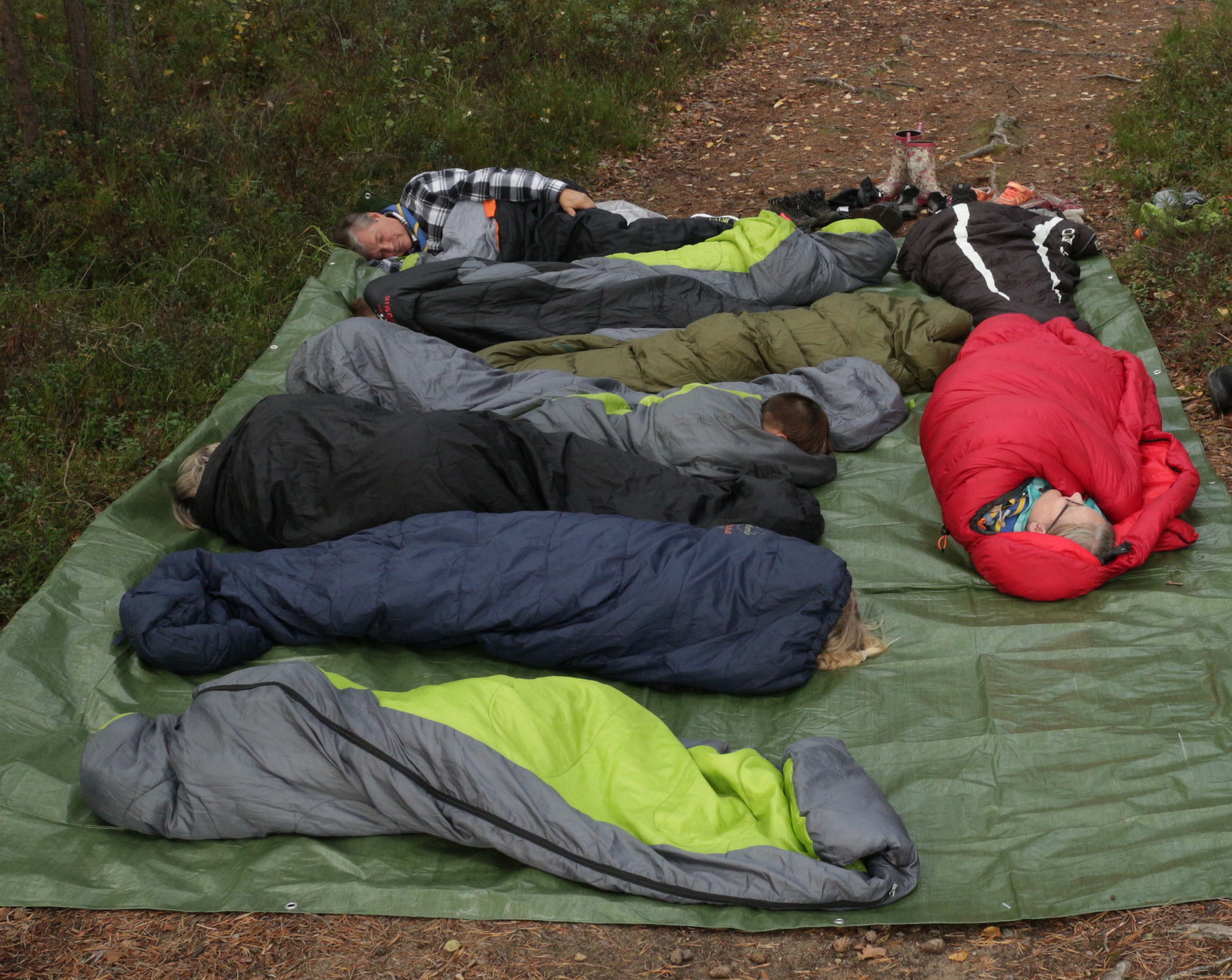The image is a color photograph taken outdoors, showing multiple people sleeping in sleeping bags laid out on a waterproof dark green tarpaulin. They are positioned horizontally across what appears to be a narrow, brown dirt or mulch walking path, likely in a forest. To the left and extending towards the back right corner of the path, there is uncut, slightly wild dark green grass tufting in places. The individuals are in various positions; some are face up, some on their sides, and one person is even face down.

The sleeping bags are varied in color: one gray and lime green, another dark blue for a blonde-haired person, a red one for a dirty blonde-haired individual, and another gray and lime green one for a man with short brown hair. There is also a military green bag, black with lime green and gray, and a black with an orange interior for an older man with salt-and-pepper hair, wearing a white and black plaid shirt and a dark blue scarf with yellow stripes. Near his feet, there is a black sleeping bag with white stripes and an older woman with salt-and-pepper hair in a red bag, wearing a cyan, dark blue, and yellow shirt. 

Alongside the sleeping individuals, there is a stack of boots and shoes to the right of the path—two pairs of black shoes and two pairs of boots, one with red ends and brown in the middle. Surrounding the scene, dark brown leaves and scattered green plants emphasize the natural, forest-like setting. This photograph captures a moment during the day, giving a glimpse into what appears to be a group of campers or potentially homeless individuals resting in an outdoor environment.